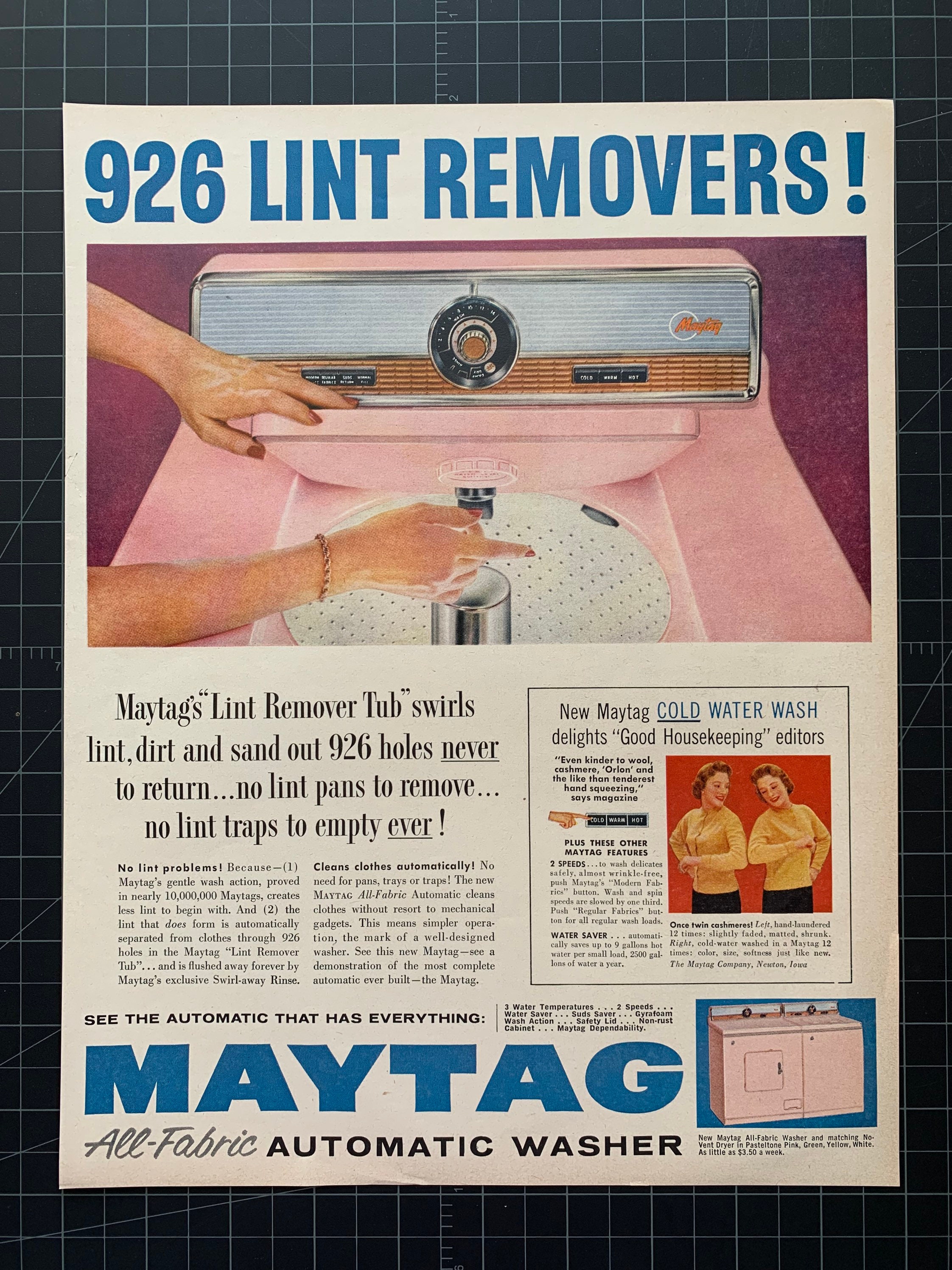This color advertisement from the 1950s or 60s, set against a black checkered background, features a Maytag All Fabric Automatic Washer. The headline boldly states "926 Lint Removers!" in blue font. The central image showcases a retro, top-loading pink washing machine with a single black control dial and black buttons with white letters, protected by a clear plastic cover. A woman’s hands, adorned with red nail polish and a rope bracelet, are seen opening the washer's lid and pointing towards the barrel, accentuating the tub's perforated design. 

The advertisement text highlights Maytag's lint remover tub technology, emphasizing: "Swirls lint, dirt, and sand out of 926 holes, never to return. No lint pans to remove, no lint traps to empty ever!" It also promotes the washer's gentle wash action, claiming it creates less lint and automatically flushes away any residual lint through its exclusive swirl away rinse system. An adjoining text box mentions a glowing review by Good Housekeeping editors, praising the washer's capability to clean even delicate fabrics like wool and cashmere.

To the right of the main image, there's a color photograph of two women, possibly twins, dressed in yellow sweaters and black slacks, standing against a red background and smiling down at their sleeves. At the bottom, another photo shows the pink washer paired with a matching dryer, reinforcing Maytag’s branding message: "See the automatic that has everything, Maytag All Fabric Automatic washer."